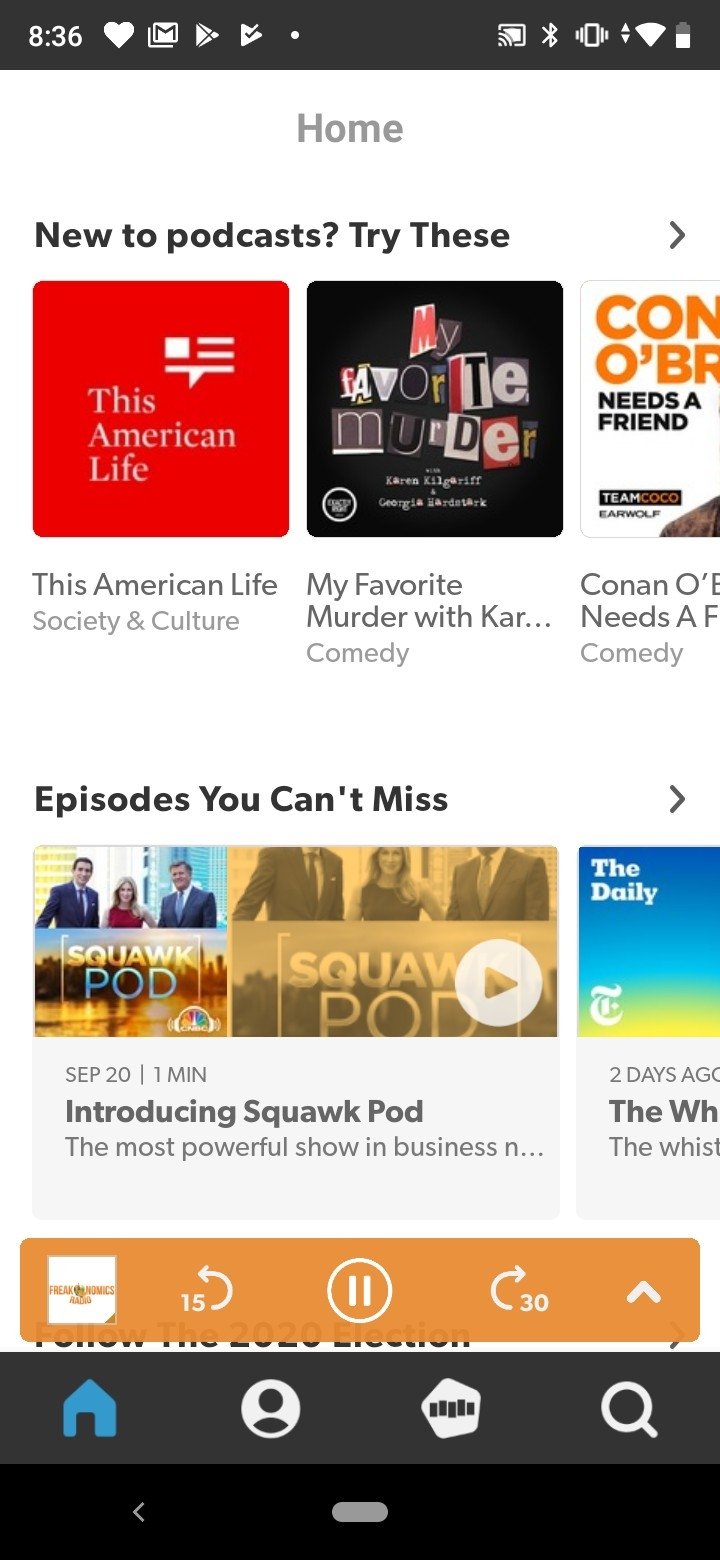The image displayed on a cell phone screen shows a strong WiFi connection and the time reads 8:36. The top of the screen features a filled white heart icon. Below this, the interface shows a gray "Home" label, followed by the text "New to podcasts? Try these" with a right-pointing arrow beside it. 

Beneath this section, various podcast recommendations are visible, starting with "The American Life" categorized under Society and Culture, highlighted in red. Next to it is "My Favorite Murder," featuring a black background with letters in different colors like red, yellow, blue, white, and gray. 

Further along is a cropped image with the text "CON OBR needs a friend," identified under Comedy. Below this category is another section titled "Episodes You Can't Miss" written in black. Featured here is "Squawk Pod," showing an image of three newscasters— two men in suits and a woman in a red dress. The image is highlighted with a gray and yellow overlay and includes a play button symbol.

Another recommended podcast, "The Daily," stands out with a blue, yellow, and green background. Below the podcast recommendations, there is an orange bar with icons, including a prominent pause button in the center. Further down, the screen shows icons for phone functions such as Home, Profile, and Search, along with a house-like icon with black lettering on a white background.